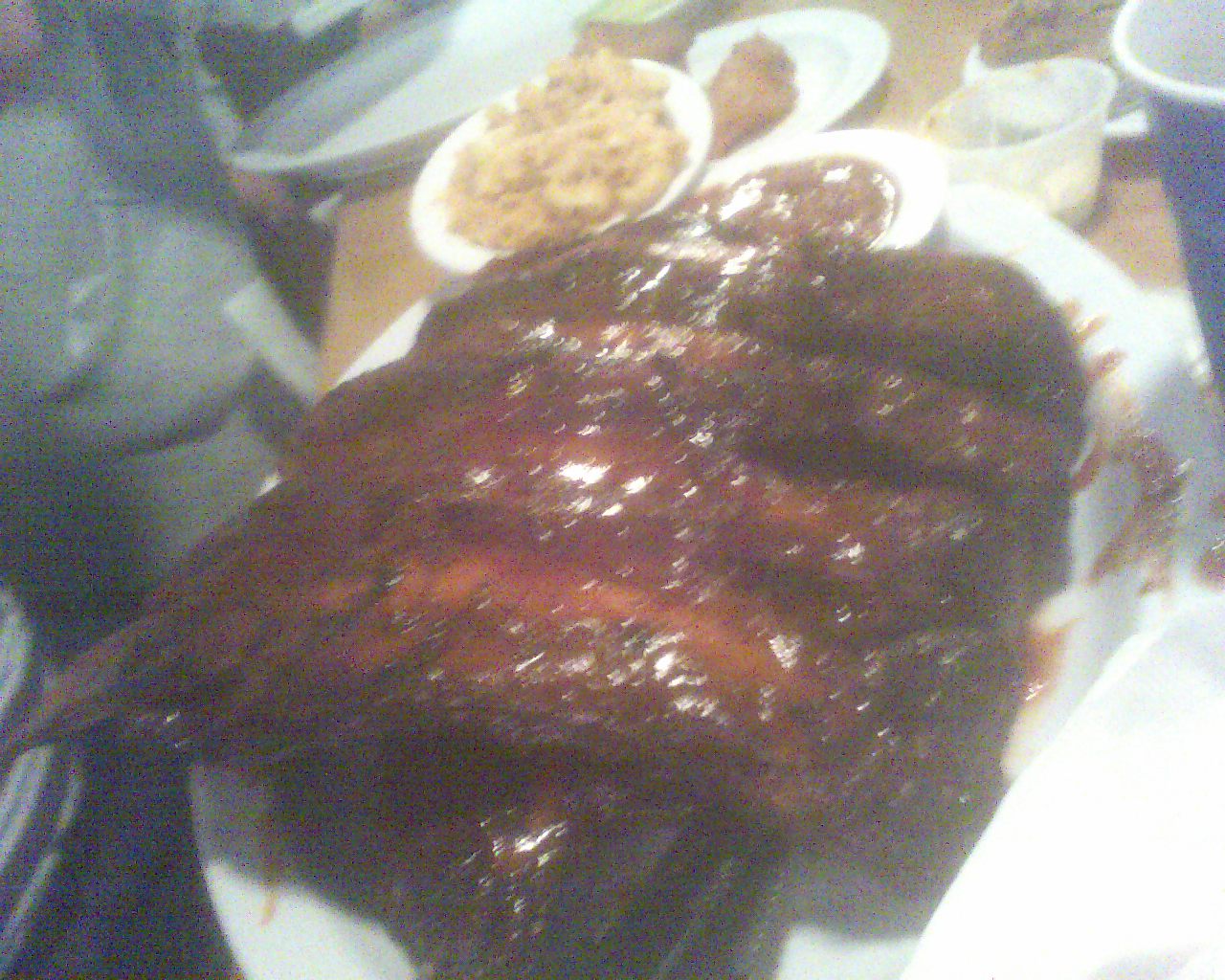This image is an out-of-focus photograph of a large stack of glazed ribs, taking up most of the frame. The ribs are drenched in a glistening, dark brown sauce, creating a wet, shiny appearance. In the foreground, there are four distinct large ribs with a mass of additional ribs beneath them. The scene is set on a brown table, where several other items are visible. 

To the left, a person with indistinguishable facial features, wearing a dark shirt with black hair, is seated. In front of the ribs, there is a white plate holding a creamy macaroni and cheese dish, and to the right of that, another small white plate with a fried chicken leg. Additionally, an empty white plate is placed in the background, alongside a clear plastic condiment cup containing a light-colored sauce. In the upper right corner, a blue disposable cup with a white interior sits, suggesting a casual dining setting. Despite the blurriness and graininess of the image, these elements suggest a hearty, finger-licking meal environment.